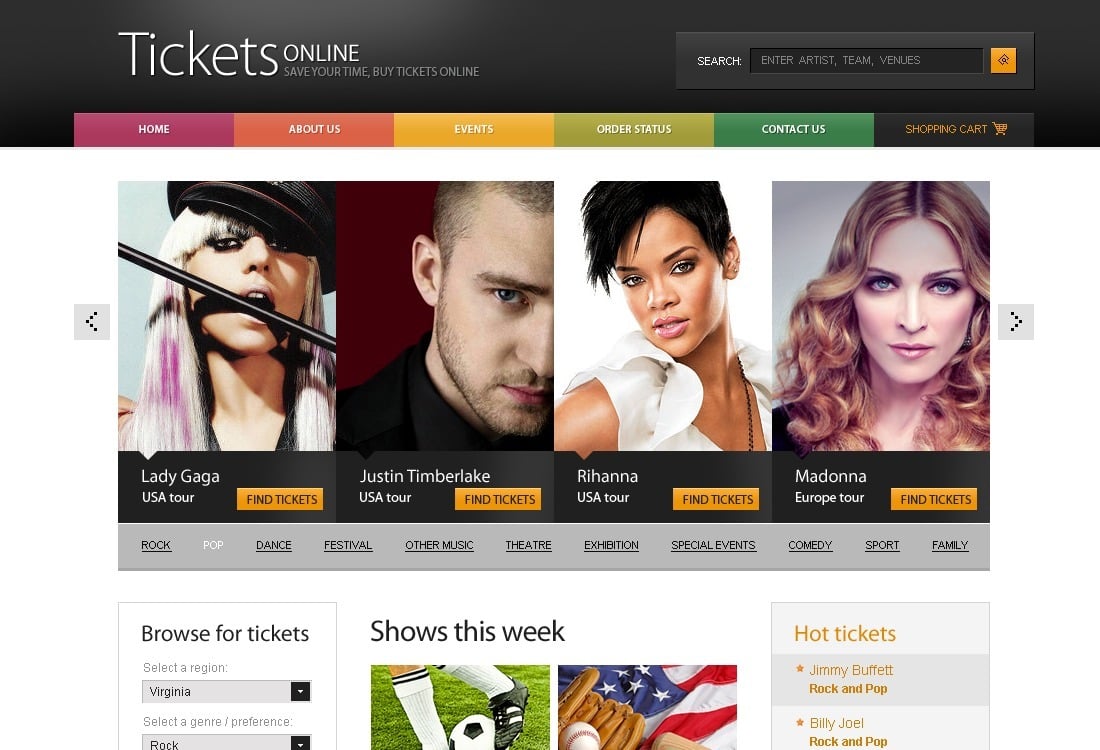The image captures a detailed view of a ticketing website's homepage. At the top, there's a dark gray navigation bar. On the left, it displays the text "Tickets" in white with a message below, "Save your time, buy tickets online." On the right side of this bar is a search box where users can 'Enter artists, teams, or venues.'

Below this, a colorful navigation menu spans horizontally across the page. It consists of six sections:
1. The first section is a red bar labeled "Home" in white letters.
2. The second section is an orange bar labeled "About Us."
3. The third section is a yellow bar labeled "Events."
4. The fourth section is a light green bar labeled "Order Status."
5. The fifth section is a darker green bar labeled "Contact Us."
6. The sixth section is a black bar labeled "Shopping Cart."

Directly beneath this navigation menu, there are four images of popular artists: Lady Gaga, Justin Timberlake, Rihanna, and Madonna. Below each artist's picture, there is an orange "Find Tickets" button.

Under these images, there is a gray bar with various categories listed for user convenience: Rock, Pop, Dance, Festival, Other Music, Theater, Exhibition, Special Events, Comedy, Sport, and Family.

On the left side of the page, there is a box titled "Browse for Tickets." This section allows users to select a region with a dropdown menu and specify their genre or preference. The default selection in this box is "Rock."

In the center of the page, there are two featured images: one of a soccer player and another of a baseball mitt and ball sitting on an American flag.

On the right side, there is a sidebar titled "Hot Tickets," featuring listings for popular events such as:
- Jimmy Buffett (Rock and Pop)
- Billy Joel (Rock and Pop)